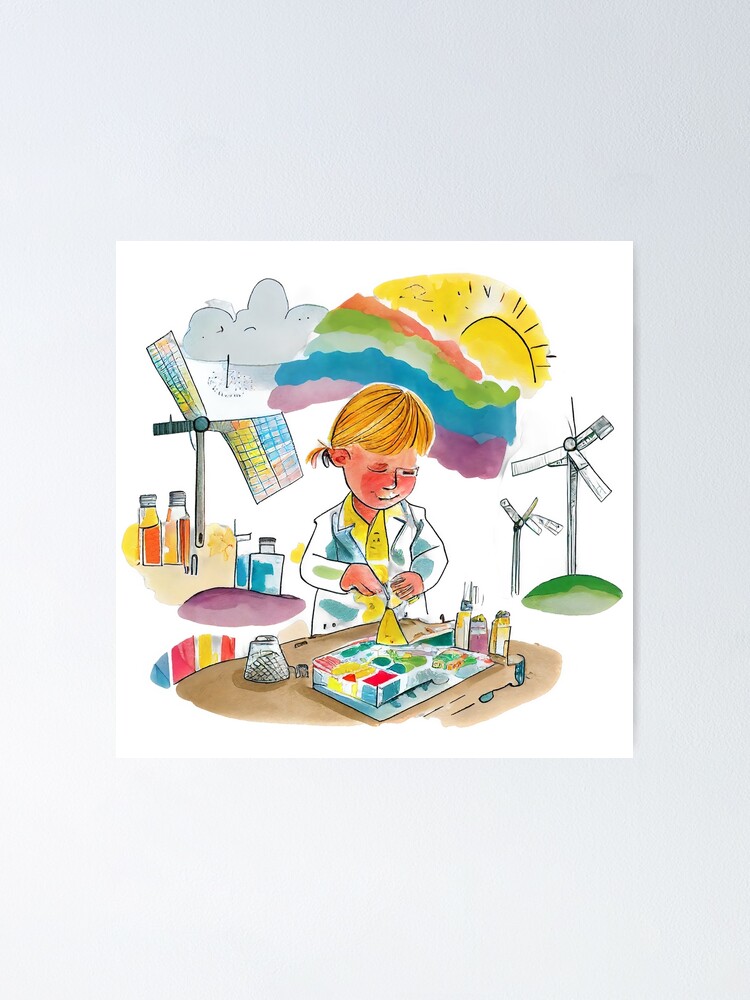This vibrant, cartoonish watercolor depicts a young girl with blonde hair, portraying an aspiring scientist amid a colorful array of objects and scenery. She stands at a table adorned with various items such as beakers, little bottles, and a divided tray filled with materials in red, yellow, blue, and green. She appears to be engaging in a science experiment with a yellow fluid, possibly painting or brushing away sand. She wears a lab coat intricately colored, adding to the playful aesthetic. Behind her, a stylized sun looms above, radiating multicolored rainbows in red, green, blue, and purple, accompanied by gray clouds. The background also features a series of whimsical windmills, some on grassy mounds and others accentuated by patches of colors including blue, yellow, and brown. Multicolored splotches decorate the scene, enhancing the overall dynamic and imaginative atmosphere.